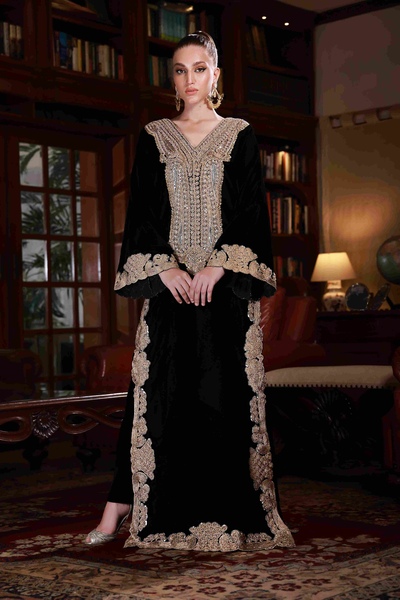The photograph, taken in portrait orientation, captures a serious-looking woman standing in an opulent study with dark mahogany bookshelves, a desk to her left, and a table with a lit lamp to her right. She appears to be Caucasian, with dark brunette or black hair pulled back into a bun. She wears a highly ornate black outfit featuring extensive gold embroidery. The dress-like garment, which includes a long skirt with gold-embroidered edges and wide sleeves, also reveals black pants beneath as she stands with one leg slightly extended. Her outfit is further complemented by elaborate gold embroidery that extends around the neck, down the middle, and along the sleeves of the garment. She accessorizes with long gold earrings and silver high-heeled shoes. The ornate elements of her attire notably include wide ornamental patterns at the shoulder and neck area, resembling a breastplate. She poses atop an oriental-style rug, adding to the image's rich, sophisticated atmosphere. Her hands are clasped in front of her, enhancing her poised and serious demeanor.